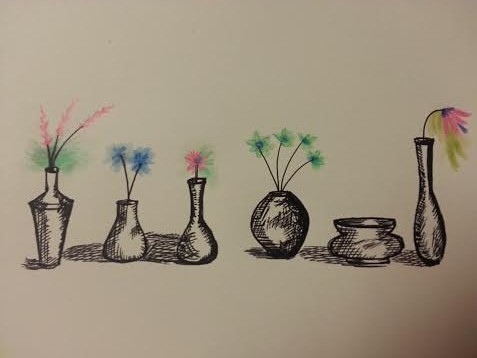The image features a slightly horizontally rectangular canvas with a dark tan background that transitions to a deep brown in the bottom right corner. Central to the composition is a meticulous pencil or charcoal drawing of several vases of varying shapes and sizes. Each vase is defined by fine, dark lines, showcasing the skillful hand of the artist. Emerging gracefully from some of these vases are delicate stems adorned with flowers in a spectrum of vibrant colors, including pinks, blues, yellows, and greens. The juxtaposition of the monochromatic vases with the vivid blooms creates a striking and harmonious contrast, bringing the still life to life against the understated backdrop.